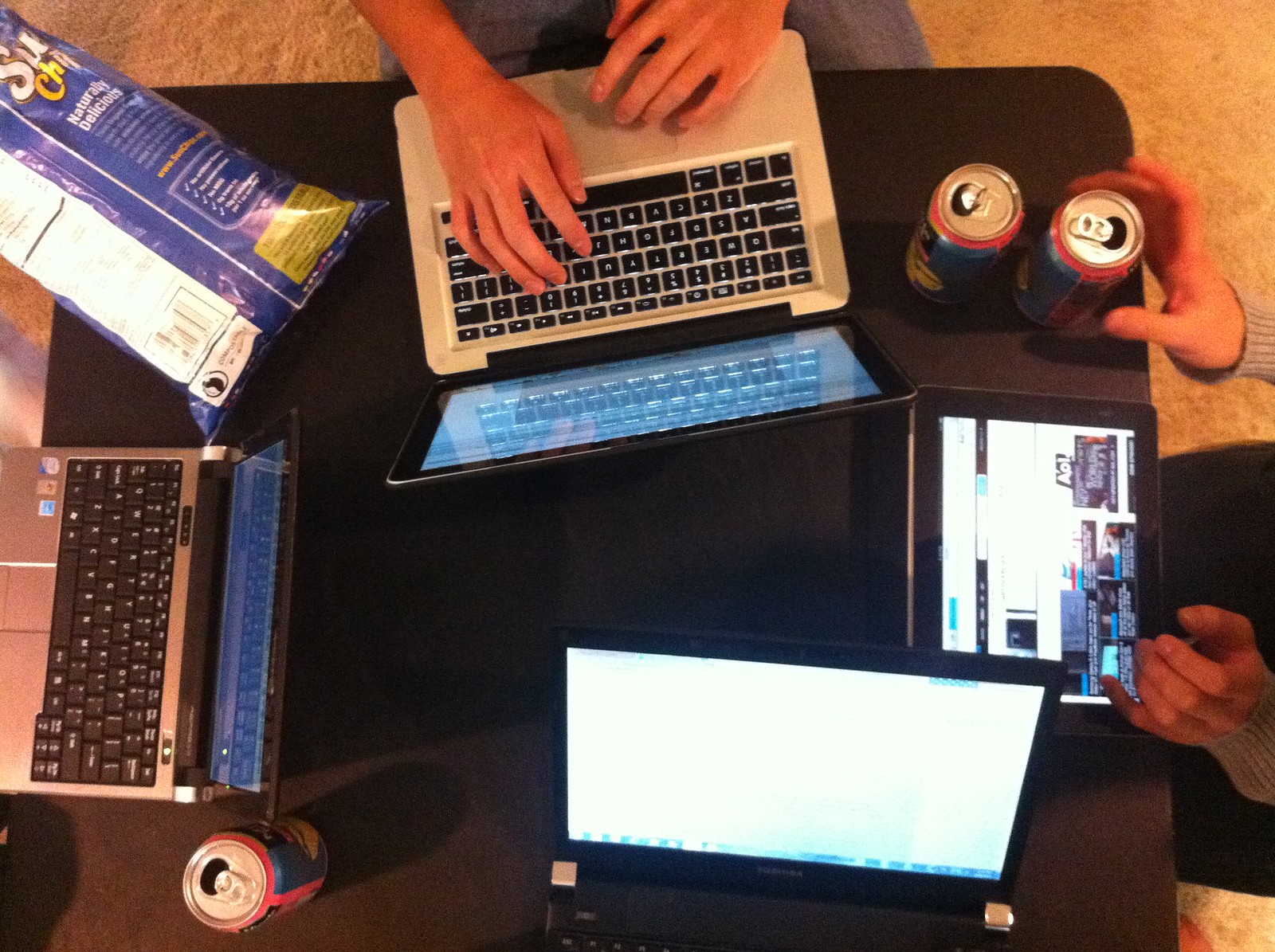This is an aerial photograph capturing a busy collaborative workspace on a black square card table, set against a creamish white, shaggy carpet. Four people are engaged with their devices, primarily laptops, in what appears to be an indoor setting. 

Starting from the top left corner, there’s a blue bag of SunChips, displaying "Naturally Delicious" and its nutrition label. A pair of hands types on a laptop with a silver keyboard and a blue screen. To the upper right, two opened blue aluminum drink cans rest on the table.

In the center, a person in blue jeans is working on a laptop with black keys and white lettering. Adjacent to this individual, on the right side, sits another person in black pants, interacting with a tablet that has a bright screen and black border. This person is also holding one of the drink cans, which can be seen mirrored across the table.

On the left side, the outline of another laptop with a visible white screen is noted. Furthermore, at the bottom center of the image, another laptop sits with a predominantly white screen, adding to the digital flurry. Lastly, at the bottom left, another top-view of an open can is visible, marking the cohesive clutter of productivity on the table.

Overall, the image captures a detailed, collaborative scene dominated by technology and snacks, emphasizing a casual yet focused work environment.